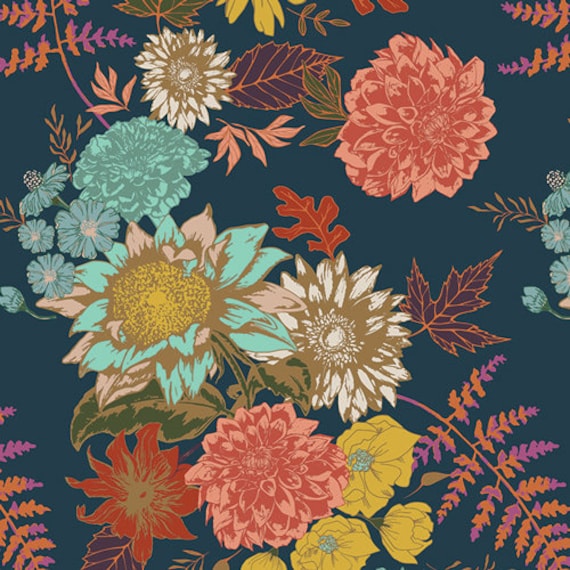The image depicts an intricate and vibrant patterned fabric or wallpaper with a dark green, possibly navy green, background. The design features a rich array of floral and leaf patterns in varying colors and shapes. Prominent flowers include a pinkish-orange blossom, a smaller white flower, a blue flower, a daisy-like bloom with pinkish and greenish leaves and a yellow center, and another flower that's white with tan accents. Additional elements in the design include multiple red and yellow flowers and a unique red-torched flower. The leaves, contributing to the lush background, appear in an array of colors such as orange, purple, and pink, with various shapes including three-pointed, regular, and fern-like forms. The entire composition exudes a harmonious yet lively aesthetic, characteristic of either a high-quality fabric or wallpaper.